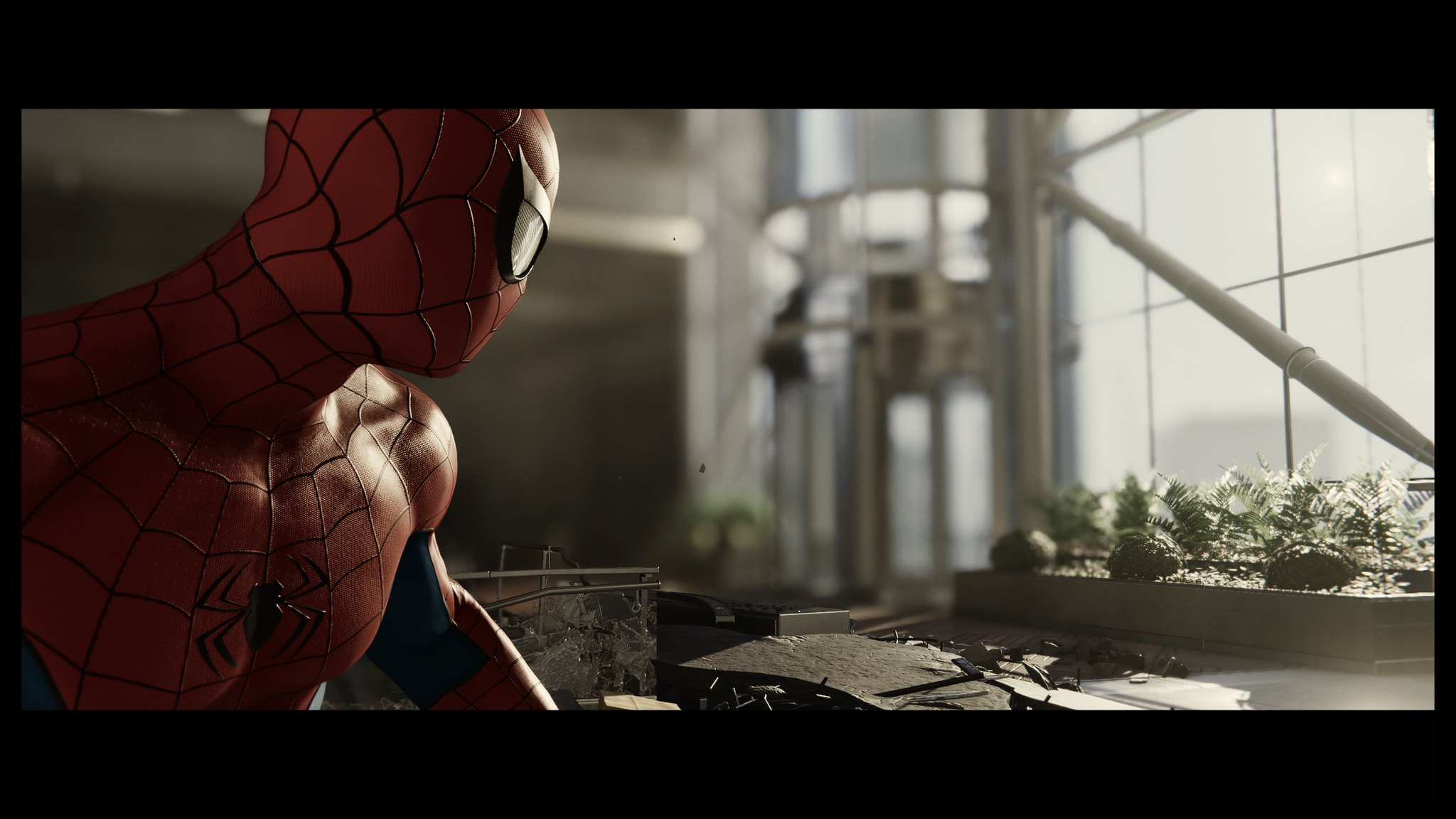A high-definition image, framed by a black border, captures a dramatic moment reminiscent of a scene from a movie or an ultra-realistic video game. Spider-Man, donned in his iconic classic spider suit, dominates the left side of the frame. He is depicted from the torso up, with his chest facing forward and his head turned as if warily glancing over his shoulder. The background reveals a chaotic atrium, littered with shattered glass and scattered debris, suggesting a recent confrontation or disaster. To the right, tall glass-paneled windows and a revolving door hint at the building's original grandeur. A planter brimming with lush ferns and decorative rocks offers a stark contrast to the surrounding wreckage, adding an element of natural beauty amidst the destruction.